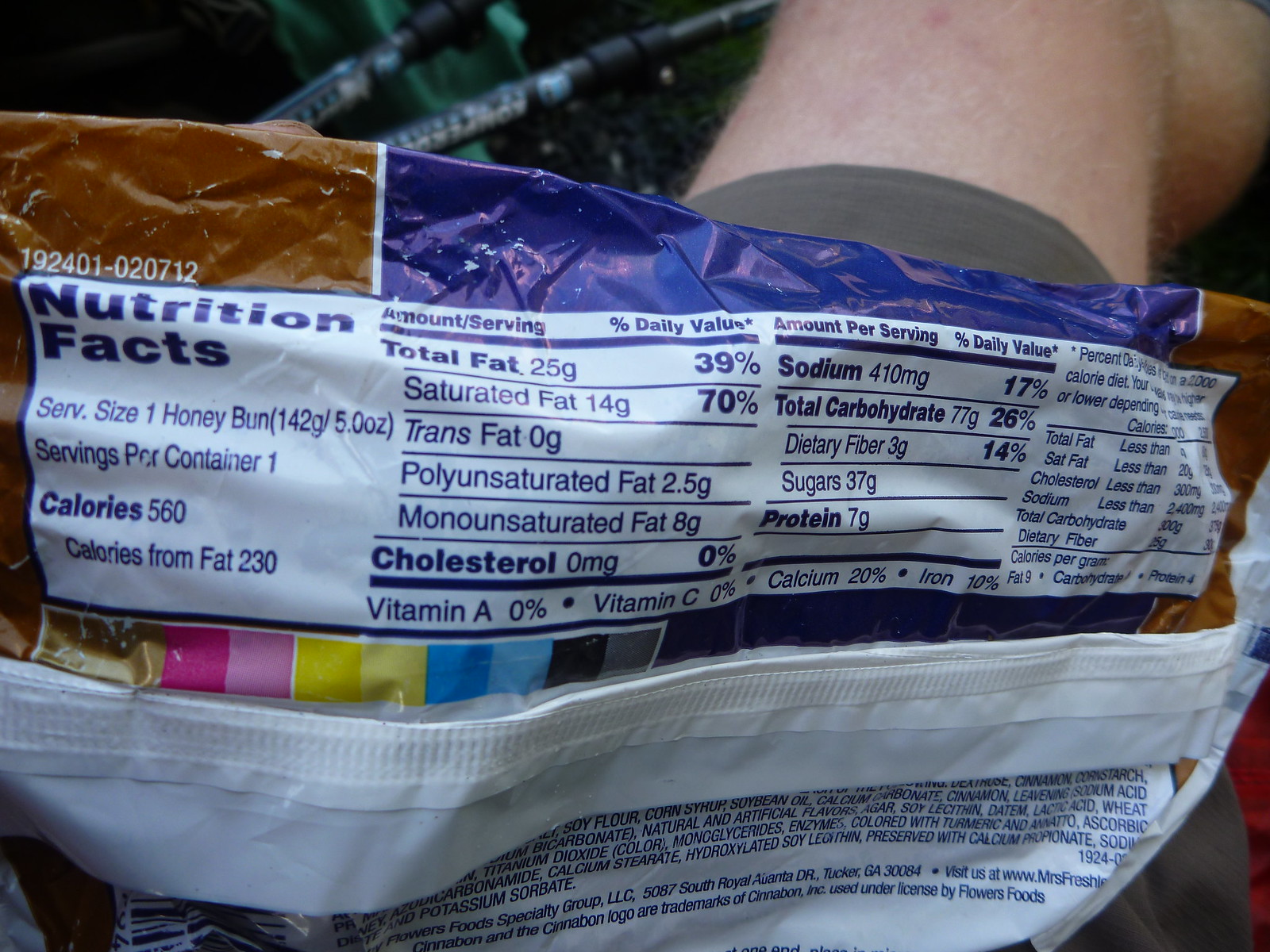A close-up photograph captures a food wrapper resting on a person’s lap. The edge of a hairy leg and gray shorts are partially visible. The wrapper is designed in shades of brown, white, and navy. A multicolored bar is visible underneath the nutrition facts, displaying squares of pink, light pink, yellow, light yellow, blue, light blue, black, and silver. The labels and nutrition facts are printed in white with navy font. The wrapper displays the following details: "Serving size: one honey bun, Servings per container: one, Calories: 560, Calories from fat: 230, Total fat: 25g, Saturated fat: 14g, Trans fat: 0g, Polyunsaturated fat: 2.5g, Monounsaturated fat: 8g, Cholesterol: 0mg, Sodium: 410mg, Total carbohydrates: 77g, Dietary fiber: 3g, Sugars: 37g, Protein: 7g." Additional nutritional values for Vitamin A, Vitamin C, Calcium, and Iron are mentioned below. Another label is positioned beside these nutritional details.